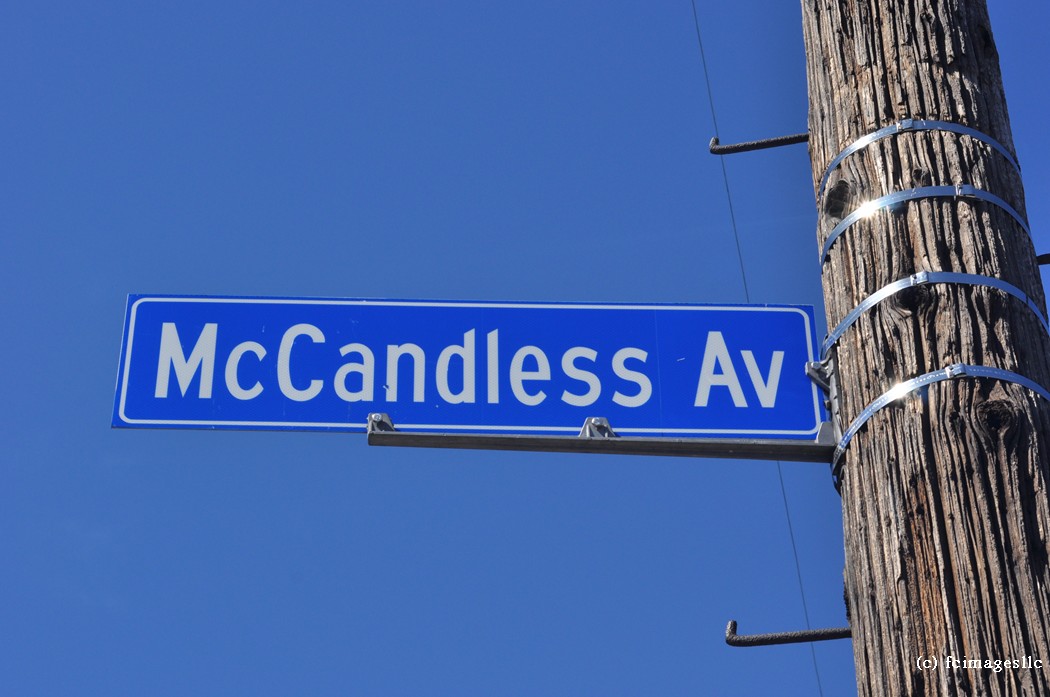This close-up photograph captures a detailed view of a street sign for McCandless Ave. The sign is a large blue rectangle, framed by a thin white border, and prominently displays "McCandless Ave" in big white letters. The sign is mounted securely on a metal arm, which is fastened to the sign at two points. This metal arm is in turn bolted onto a weathered wooden utility pole, characterized by visible knots and textures in the wood. 

The pole is reinforced with four evenly spaced silver metal straps, numbered from top to bottom, which tightly girdle the trunk of the pole. A power line stretches diagonally from the upper part of the image downwards, cutting across the pristine, cloudless blue sky that serves as a backdrop for the composition. In the bottom right corner of the image, there is a small white copyright notice along with a tiny name, adding a subtle but discernible mark of authenticity.